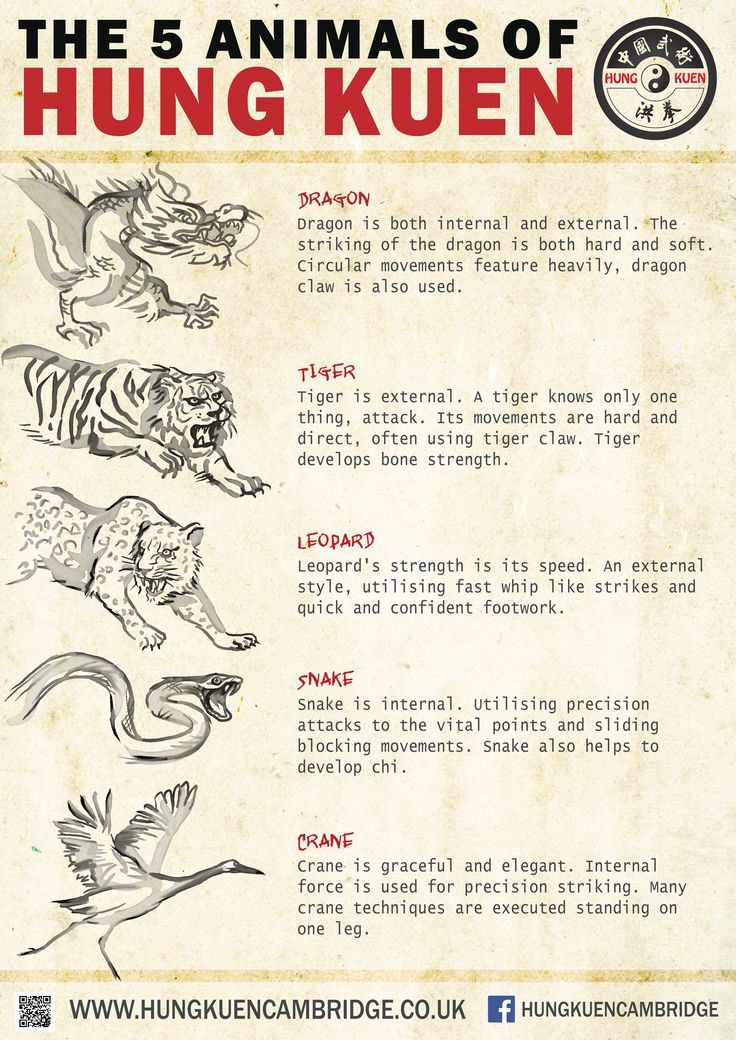The image is a detailed and visually striking infographic, possibly a scan of a poster or a screenshot from a website, depicting "The Five Animals of Hung Kuen" martial arts. At the top, the title is prominently displayed with "The Five Animals of" written in black and "Hung Kuen" in red. The infographic features black and white Chinese-style illustrations of a dragon, tiger, leopard, snake, and crane, aligned vertically down the left side. 

Each animal has a dedicated section with a detailed paragraph explaining its unique characteristics and attributes in the art of Hung Kuen. The dragon is represented with both internal and external techniques, emphasizing soft and hard circular movements and the use of the dragon claw. The tiger is described as purely external, focusing on direct and powerful attacks that develop bone strength, often utilizing the tiger claw. The leopard is noted for its speed and external style, characterized by fast, whip-like strikes and agile footwork. The snake is an internal style, using precision attacks on vital points and sliding blocks to develop chi. 

The crane is also depicted as one of the five animals, although detailed information about its characteristics was not specified in the earlier descriptions. At the very bottom of the infographic, there are additional details including a website and social media links—hongquincambridge.co.uk and a Facebook page for Hung Kuen Cambridge, reinforcing the digital or online nature of the source.